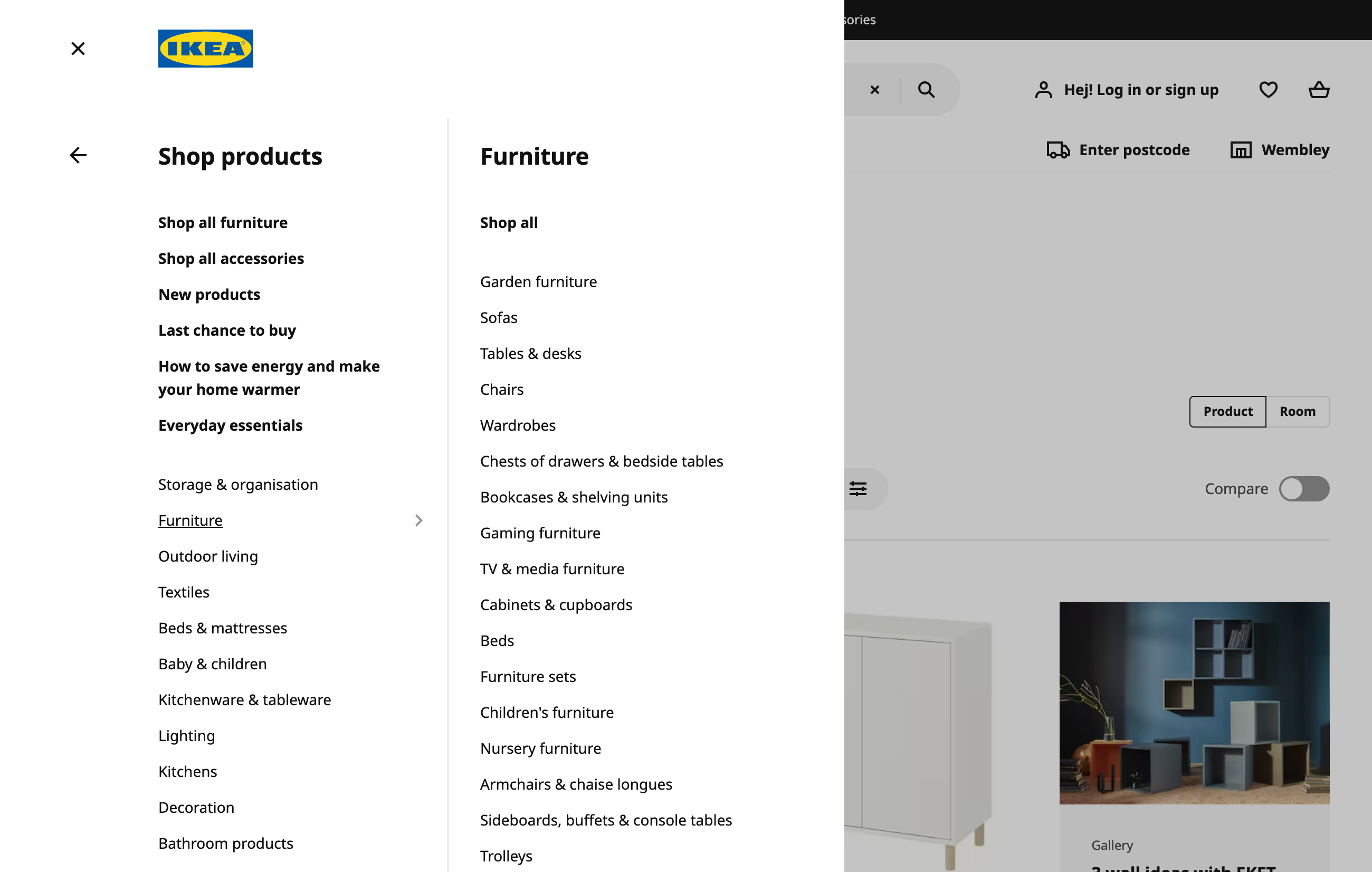Detailed Descriptive Caption:

This screenshot captures a specific section of an Ikea website, presented in Swedish. On the left-hand side of the image, we observe two vertical columns in white. In the top left corner, the prominent blue and yellow Ikea logo is displayed, with the word "Ikea" in red letters inside it. Below the logo, the left column begins with a header that says "Shop Products," followed by an extensive list of shopping categories, including "Shop all furniture," "Shop all accessories," "New products," "Last chance to buy," "How to save energy and make your home warmer," "Everyday essentials," "Storage and organization," and various others such as "Furniture," "Outdoor living," "Textiles," "Beds and mattresses," "Baby and children," "Kitchenware and tableware," "Lighting," "Kitchens," "Decoration," and "Bathroom products."

On the right-hand side, next to the left column, we see another column specifically dedicated to furniture. At the top, it has the header "Furniture," followed by a "Shop all" option. This column enumerates several categories of furniture items, such as "Garden furniture," "Sofas," "Tables and desks," "Chairs," "Wardrobes," "Chests of drawers and bedside tables," "Bookcases and shelving units," "Gaming furniture," "TV and media furniture," "Cabinets and cupboards," "Beds," "Furniture sets," "Children's furniture," "Nursery furniture," "Armchairs and chaise lounges," "Sideboards, buffets, and console tables," and "Trolleys."

The main part of the webpage, located to the far right, shows additional page details. In the top right corner, there is a login prompt that says "Hey, log in or sign up," with the greeting "Hey" written as "HÄJ," signifying the website's Swedish language setting. Below this, options are available to enter a postcode and select the location "Wembley." At the bottom of the webpage section visible in the screenshot, there is an image within a gallery, depicting a blue wall adorned with various stacking items.

This thorough description captures the structure and content of the web page section depicted in the screenshot, emphasizing its detailed layout and functional design elements typical of Ikea.